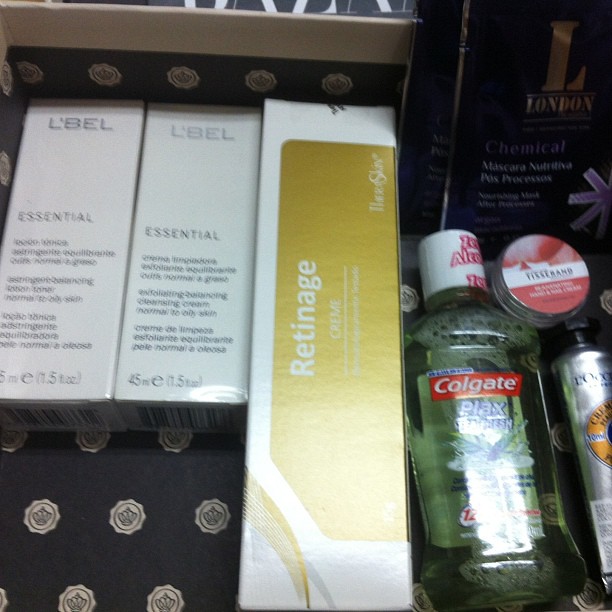In this photograph, we see an assortment of beauty products arranged inside a decorative box. The box, featuring a white edge with an interior lined in black paper, showcases a repeating logo of black crowns encircled in light gray or tan. Starting from the upper left, two identical white boxes prominently display "L'BEL Essential" in black text, though other details are too blurry to discern. To the right, a rectangular box with a predominantly white background and a central gold banner reads "Retin-Age Cream." Below and to the right of this is a clear container of Colgate Plax mouthwash, containing green liquid and topped with a white cap. Next to it sits a small cylinder labeled "First Band," displaying a white banner over a pink background. Additionally, a noticeable silver tube with a black cap is positioned at the bottom right. In the upper right corner, two purple packets with gold text read "London Chemical" partially obscured by blur. The arrangement and variety of products suggest an organized display of someone's toiletries for easy access.